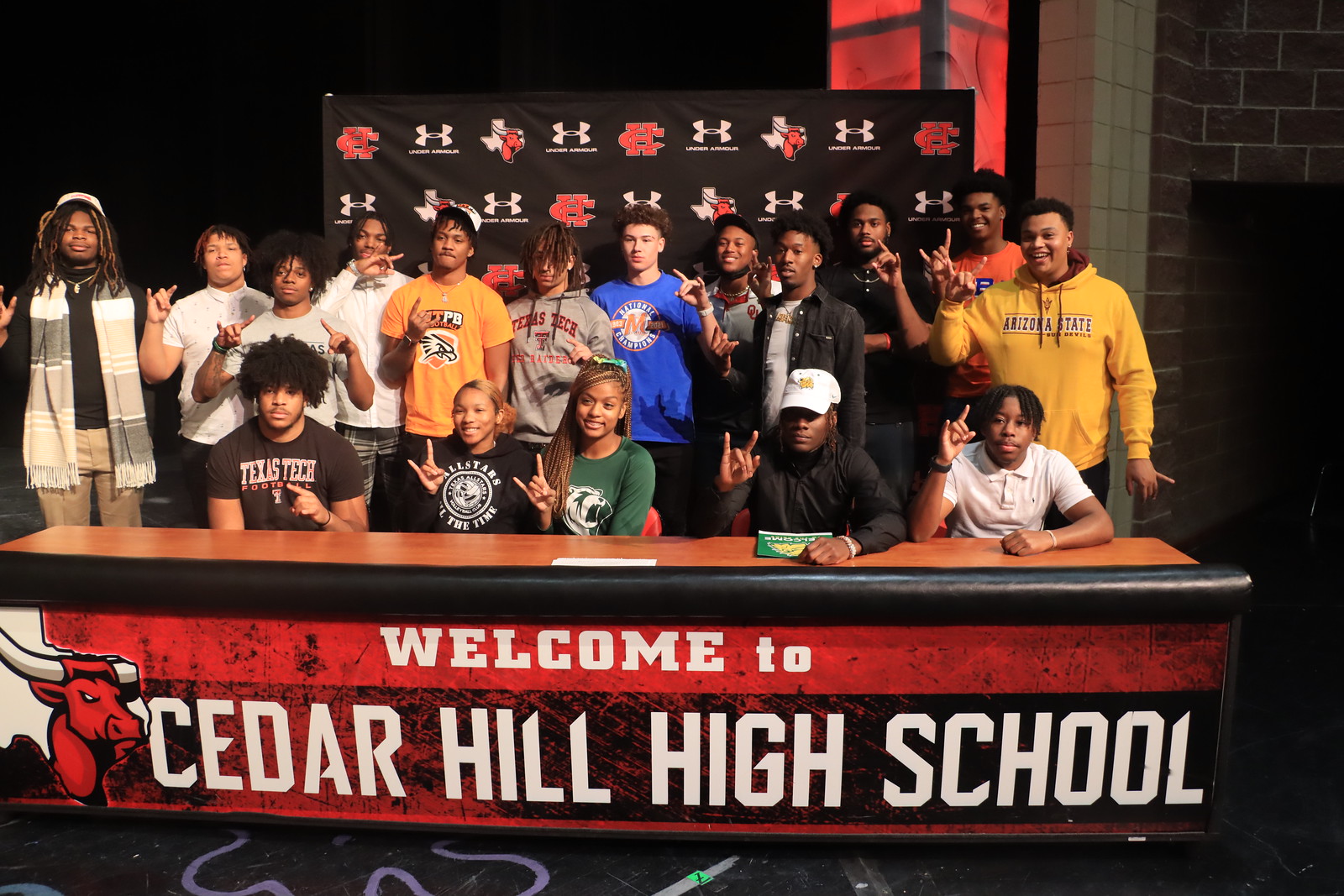This photograph, taken inside a building at Cedar Hill High School, features a group of about 20 students posing together. They are both sitting and standing behind a long table adorned with a red banner that reads "Welcome to Cedar Hill High School" in white font, with a red bull situated on the left side of the banner. In the front row, two females are seated at the table, making a hand sign resembling horns. The remaining students stand behind them, all contributing to the group's energetic pose by making the same hand sign. Most of the students are African American males, with one Caucasian individual present. They are dressed in a mix of hoodies and t-shirts, suitable for varying weather conditions. The background features imagery from Under Armour on the left side, while the right side displays a brick wall leading to a dark corridor, contrasting against a black backdrop. The floor beneath them also has some drawings, adding to the setting's detailed environment.